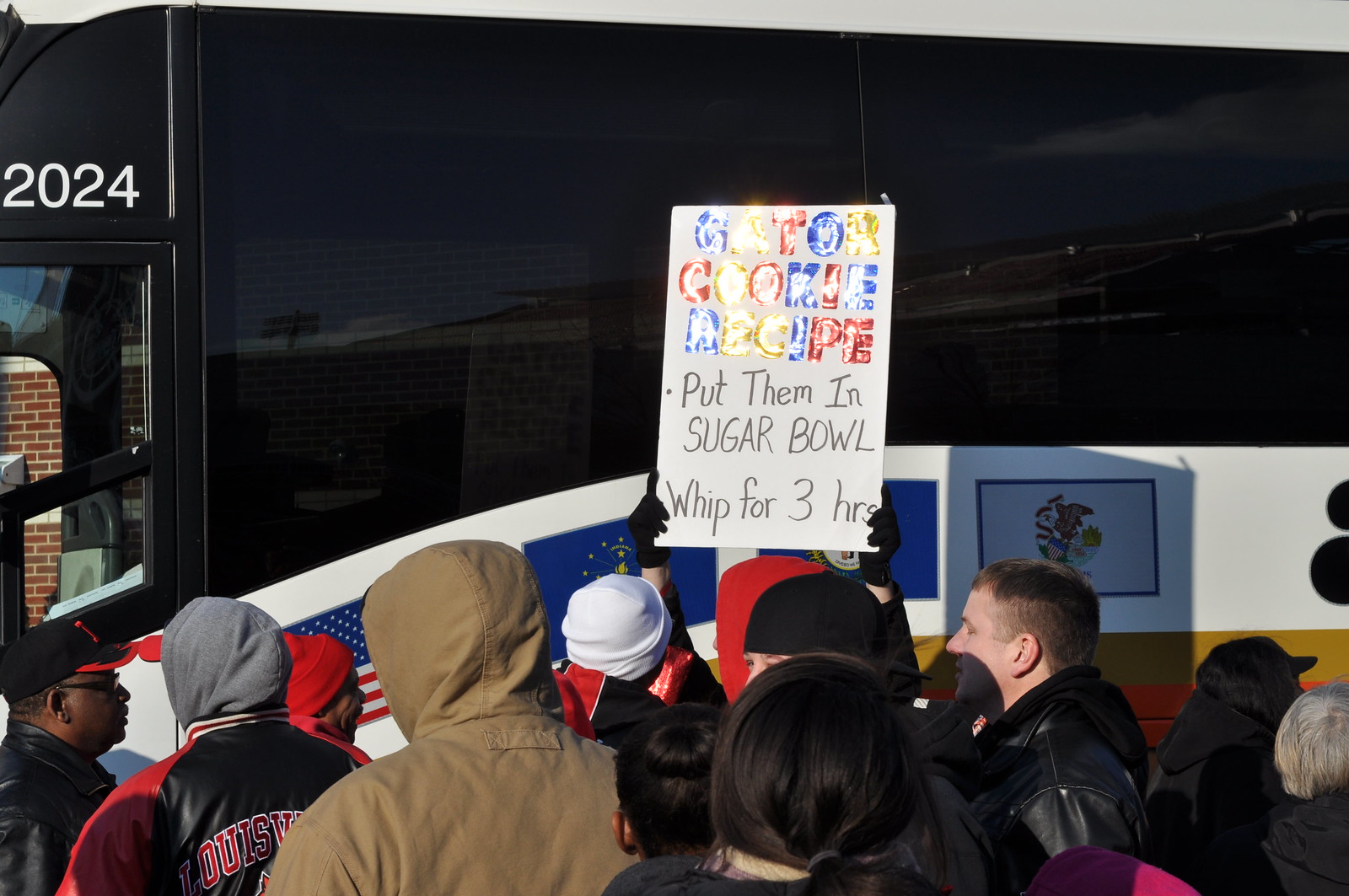In this color photograph, a large black bus dominates the background, featuring bold white numbers "2024" at the top, just above the door. The bus has distinct design elements, including a white curved stripe across its midsection, flanked by smaller gold and red bars. Along its side, several flags, including those of the United States and the European Union, are visible, though some details of the flags are indistinct.

In the foreground, a dense crowd occupies the lower part of the image. The individuals are dressed in jackets, parkas, ball caps, and knitted caps, indicating a cold environment. Many have their hoods pulled up and are wearing gloves. Central to the photograph is a person, barely visible, holding a rectangular poster board from the bottom corners. The sign reads, in thick, alternating blue, yellow, and red letters: "Gator Cookie Recipe." Below that, handwritten in black sharpie, it instructs: "Put them in sugar bowl, whip for three hours." The sun's reflection partially obscures the top part of the sign, adding a glare that makes some letters less legible. The overall scene has a somewhat static feel, as if the crowd is waiting for an event to unfold.